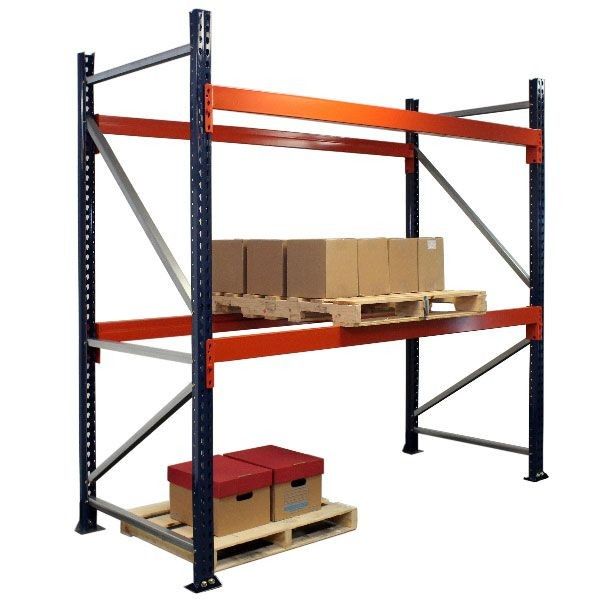This is a professionally lit and photographed color image, seemingly from a website, showcasing an industrial shelving unit in a warehouse setting. The shelving unit is constructed from black steel uprights with small holes for adjustable height, and bright orange steel crossbars, which create two levels of storage. The photograph's white background highlights the shelving, drawing attention to the detailed components.

On the lower level, the orange crossbars support a light wooden pallet loaded with a variety of rectangular brown cardboard boxes, some featuring unreadable blue text. Underneath this level, another wooden pallet sits on the floor to the left, holding two additional cardboard boxes with distinct red lids and handholds. This combination of colors, including touches of gray and blue, along with the meticulous arrangement of the elements, suggests a professionally staged and photographed setup, ideal for advertising the utility and organization potential of the shelving unit.